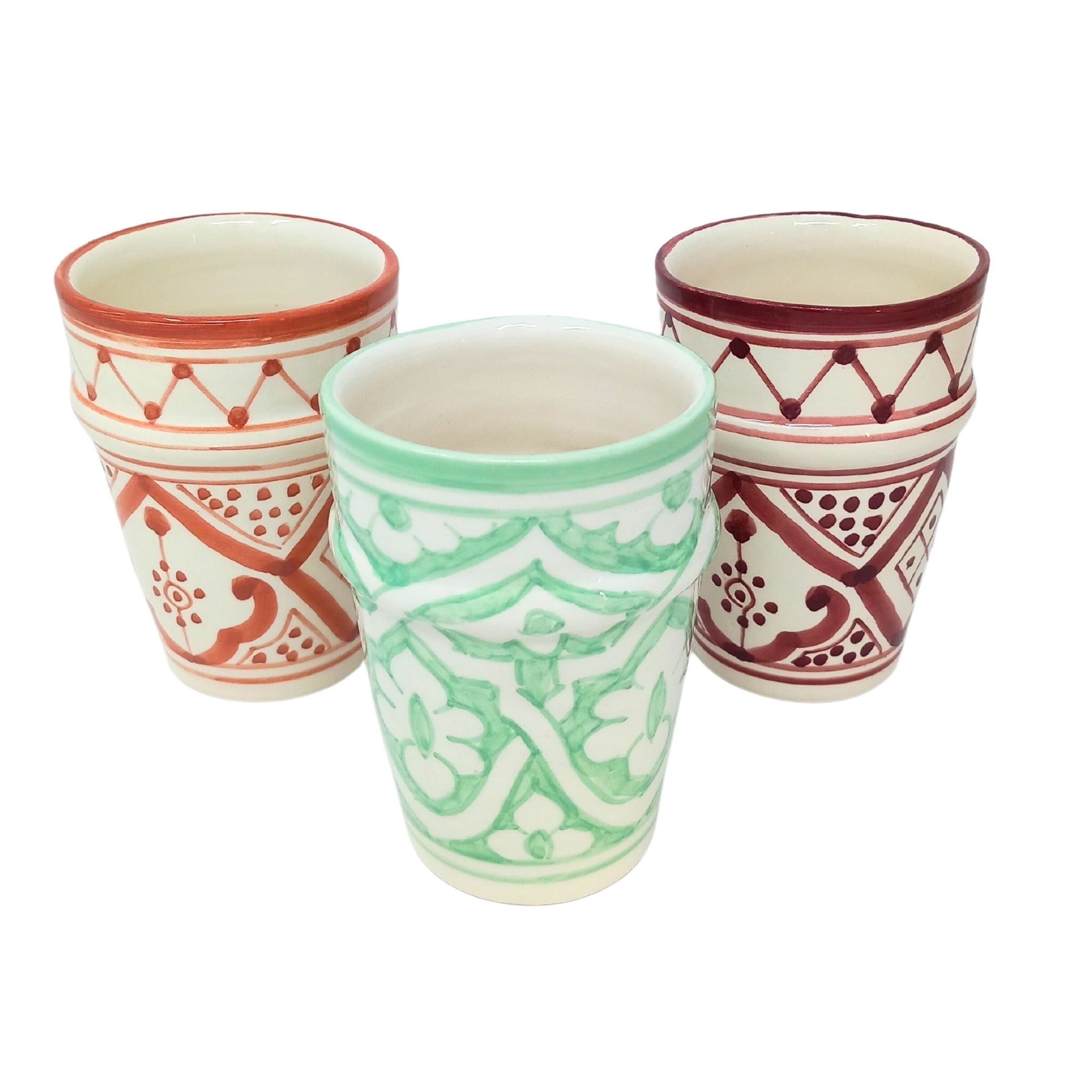The image features three intricately designed pottery cups, each with a unique color and pattern. These cups are crafted with a narrower base that expands towards the top, where a distinctive lip projects out three-quarters of the way up, facilitating an easier grip.

Each cup is individually colored—one in vibrant orange, another in a rich maroon, and the third in a deep green. The orange and maroon cups are positioned in the back and feature a drum-like design on their upper sections. This design consists of dots interconnected by a zigzagging line, creating a rhythmic pattern. In contrast, the green cup at the front showcases a continuous floral motif that gracefully extends over the lip. The thick, swirling lines interconnect to form shapes reminiscent of the peak of an 'A', adding an elegant touch to its surface.

All three cups are displayed on a pristine white surface against a stark white background, emphasizing their detailed craftsmanship and vivid colors.